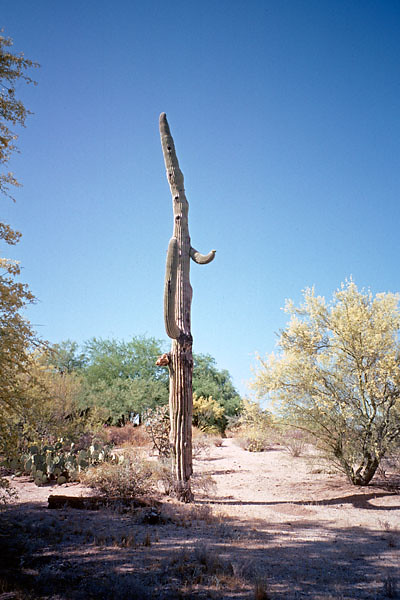The photograph captures a serene desert scene under a cloudless, blue sky. The primary subject is a towering cactus that stands prominently in the center, stretching to a striking height of about nine to twelve feet. Unusually shaped, the cactus has a slender, vertical trunk with two protrusions mimicking human arms—one held out in front on the left and another positioned towards the waist on the right. Four distinct dark circles line the upper half, and the cactus tapers to a pointed top. The ground is a characteristic light tan, typical of desert terrain, dotted with dry grass and mostly bare. To the right side of the image, a small shrub or tree with light green-yellow leaves adds a splash of color. In the background, various smaller cacti and low-lying desert trees are visible, contributing to the arid landscape. A trail-like open area devoid of any pavement weaves through the scene, suggesting a natural path through the desert. The photograph is bathed in daylight, likely taken in the early evening.